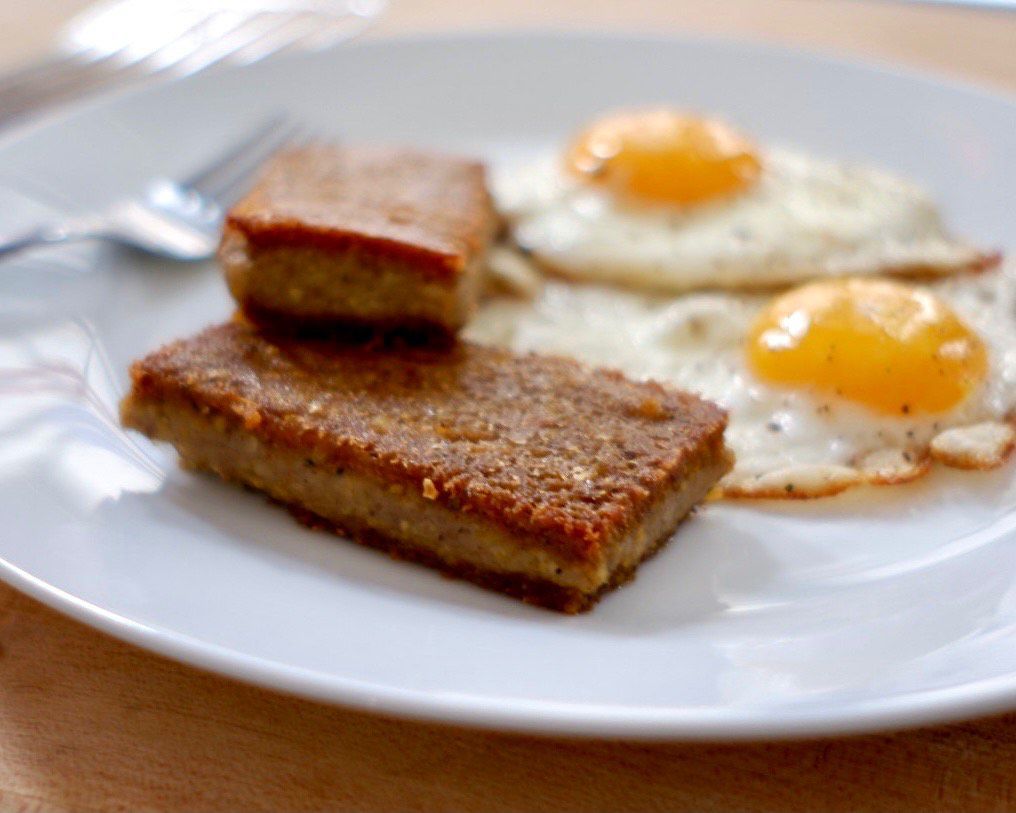The image features a close-up of a breakfast plate set on a brown wooden table. On the white, round plate, there are two sunny-side-up fried eggs with partially cooked yolks, seasoned with a sprinkling of black pepper. To the left of the eggs lies a pair of rectangular, granola bar-like toast pieces. The top surfaces of these toast pieces have a moist reddish hue, making them appear somewhat unusual. A metal fork is positioned on the left side of the plate, resting partially on it and on the table. The focus of the photograph is sharp on the breakfast foods, particularly emphasizing the detailed textures of the eggs and the distinct appearance of the toast, while the surrounding elements, including the fork and the table, remain discernibly visible.